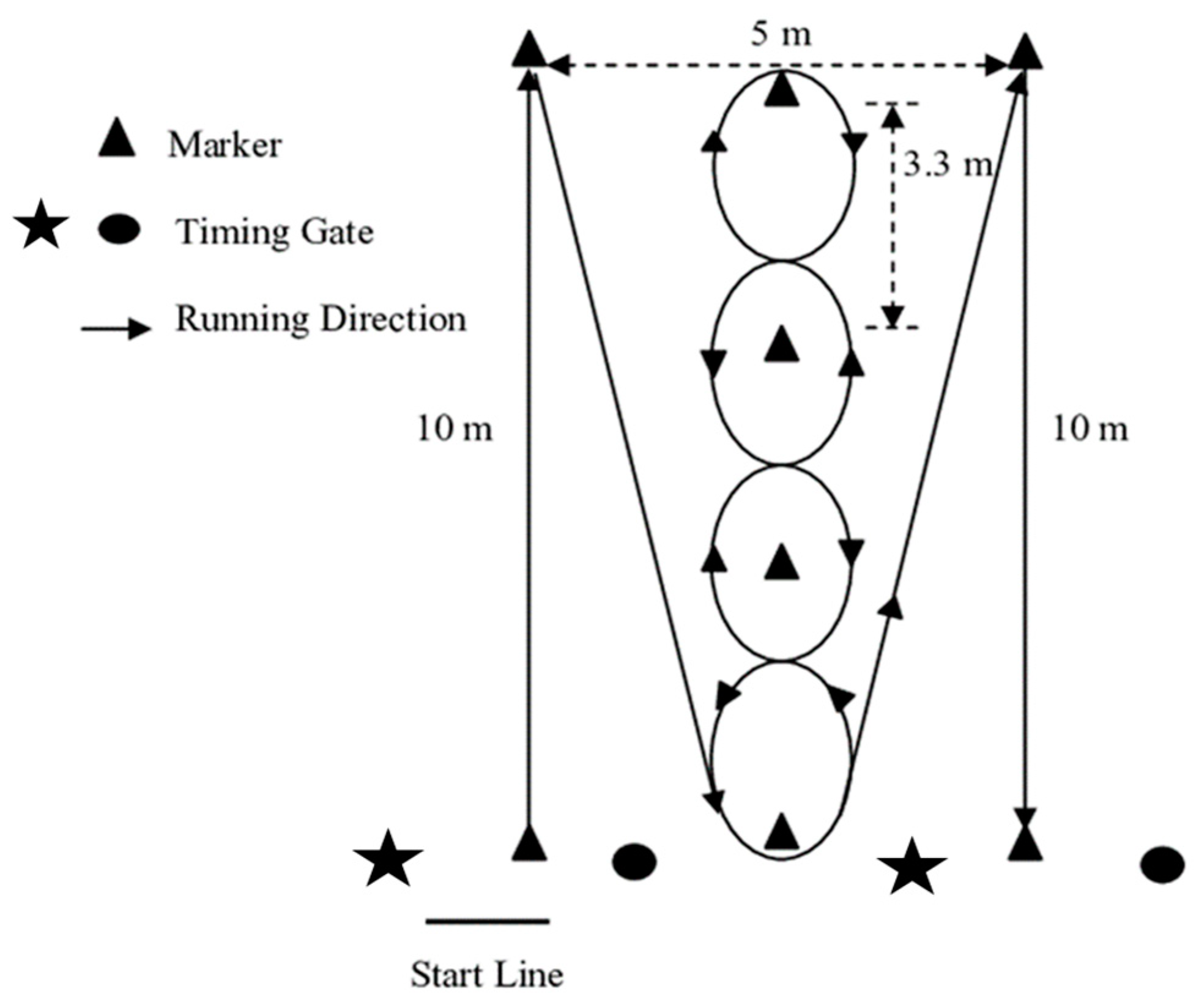This detailed diagram, presented in black ink on a white background, appears to illustrate a measurement or tracking system. The primary diagram occupies the right side, featuring various geometric shapes and lines. At the bottom left, a black triangle anchors a vertical line ascending to a black arrow. Rightward, a black oval leads to a black star, followed by another triangle with a similar line and arrow configuration. A black arrow at the bottom points back to the triangle.

Connecting these figures is a black dotted line that spans the top, intersected with small arrows at each endpoint. Above this line, the notation reads "5M." Central to the design, a continuous line originates from the top-left arrow, descends and curves rightward at the bottom, looping upward to the top-right arrow. This loop encloses several ovals stacked vertically, each marked with an upwards-pointing black triangle. Outside these ovals, additional triangles point both up and down.

To the diagram's bottom left, a short horizontal line denotes the "start line," marked below by another line. A black star is situated above and to the left. Vertical scales flanking the design show "10M," indicating a 10-meter span, and a right-side dotted line measures "3.3M" between ovals. 

An upper-left key explains the symbols: triangles stand for markers, stars and ovals for timing gates, and arrows indicate the running direction. This infographic likely outlines a spatial arrangement, possibly for a timed navigation course or movement tracking system.